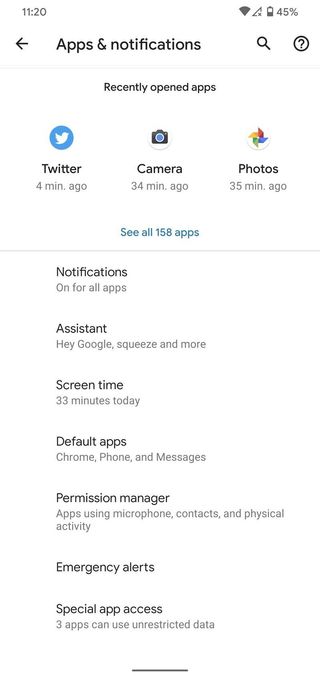The image depicts the "Apps & Notifications" settings screen on an Android phone in light mode, featuring a clean white background. At the top of the screen, there's a section titled "Recently Opened Apps," listing Twitter, Camera, and Photos with the respective usage times: Twitter (4 minutes ago), Camera (34 minutes ago), and Photos (35 minutes ago). Below this list is an option labeled "See all 158 apps."

Further down, there's an "Options" section offering several settings: "Notifications," "Assistant," "Screen Time," "Default Apps," "Permission Manager," "Emergency Alerts," and "Special App Access." The "Special App Access" section reveals that three apps have unrestricted data usage. The "Permission Manager" provides details on apps that access the microphone, contacts, physical activity, among other permissions.

The "Screen Time" display indicates the phone has been used for 33 minutes today, while the "Notifications" setting is turned on for all apps. In the notification area, the phone shows 45% battery life remaining, no cellular signal, but full Wi-Fi connectivity. Users can adjust app permissions, manage notifications, and configure other app-related settings from this screen.